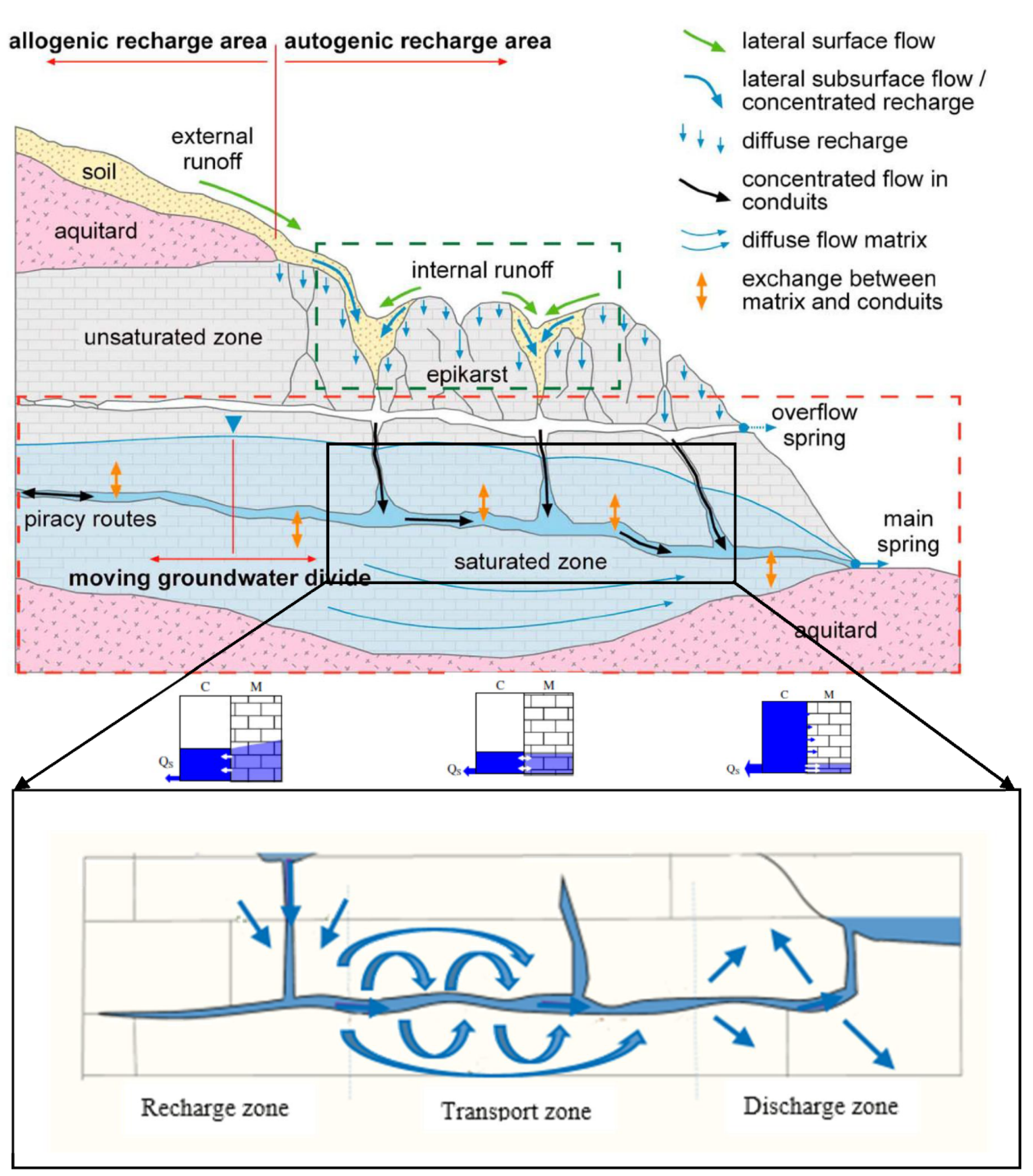This scientific diagram, likely from a textbook, illustrates the process of groundwater recharge and flow within both allogenic and autogenic recharge areas. At the very top, the chart identifies these recharge areas, depicting the internal structure of a hillside with various layers. The diagram includes layers such as soil, aquitard, and an unsaturated zone, along with a moving groundwater divide. Arrows indicate the direction of water movement, showing lateral surface flow, lateral subsurface flow, internal runoff, and diffuse and concentrated flows through conduits. The top-right corner features a legend with symbols for these flows, mapped out in green, blue, black, and orange. The lower section of the diagram breaks down the process further into three zones: the recharge zone, transport zone, and discharge zone. Collectively, this detailed chart delineates the complex interactions between soil, water, and geological formations, highlighting the movement of water from infiltration to discharge.